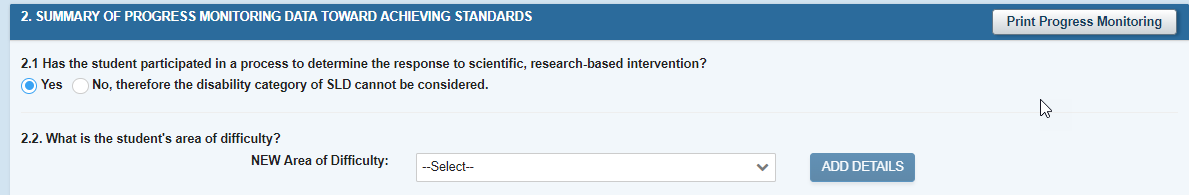The image is a screenshot of a notification on a webpage with a predominant blue color scheme. The background is a solid blue, while a lighter blue box overlays it. At the top of this lighter box is a medium to dark blue bar, featuring white, all-caps text in a bold sans-serif font that reads: "SUMMARY OF PROGRESS MONITORING DATA TOWARD ACHIEVING STANDARDS." On the right side of this bar, there is a white button with blue text that says "PRINT PROGRESS MONITORING."

Below this bar, within the lighter blue box, there is black sans-serif text that reads: "2.1 Has the student participated in a process to determine the response to scientific, research-based intervention?" Beneath this question are two bullet-point options. The first option, which is selected, reads "Yes." The second option reads, "No, therefore the disability category of SLD cannot be considered."

Following this, there is another heading: "2.2 What is the student's area of difficulty?" Under this heading, it says "New area of difficulty," accompanied by a drop-down menu labeled "Select" and a blue button that reads "Add Details."